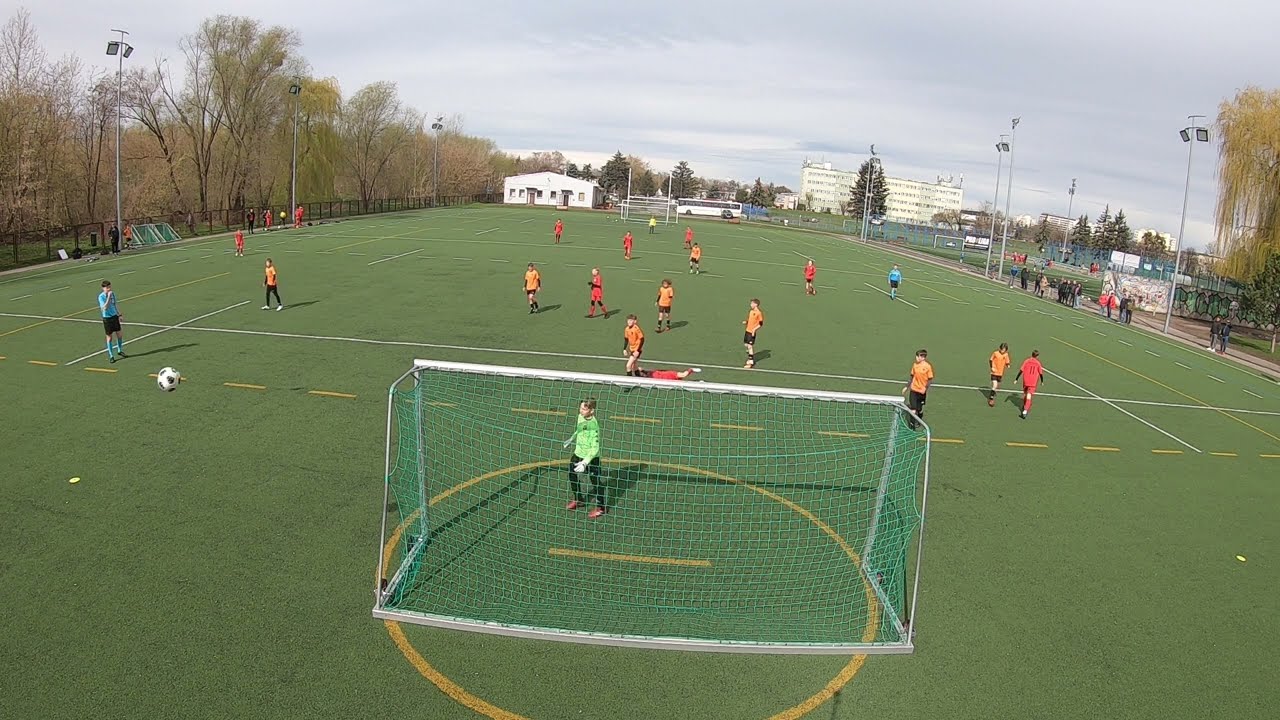The image depicts a large soccer field under an overcast sky, featuring predominantly gray clouds. In the distant background, there's a white building with indistinct details. The field itself is green turf marked with white and yellow lines, indicating it is used for multiple sports. 

Scattered across the field are several players, suggesting a youth soccer game. One team is dressed in orange jerseys and black shorts, while the other team sports red jerseys and black shorts. The goalie stands near the goalpost, wearing a lime green long-sleeve shirt and black pants, facing toward the goal. The soccer ball is located on the left-hand side of the goal, moving towards the area where the goalie is positioned.

Spectators, likely parents, are seen on either side of the field, implying that there aren't any bleachers available, and they might have brought their own chairs. Tall light posts stand on both the right and left sides of the field, although they aren’t in use during the daylight. The field is encircled by trees, adding a natural border, and there are various yellow dotted lines and markings for different sports.

Notably, the scene includes a large bus, possibly used to transport one of the teams from another part of the city. Despite the absence of text in the image, all these elements combine to suggest an organized youth soccer match in progress.